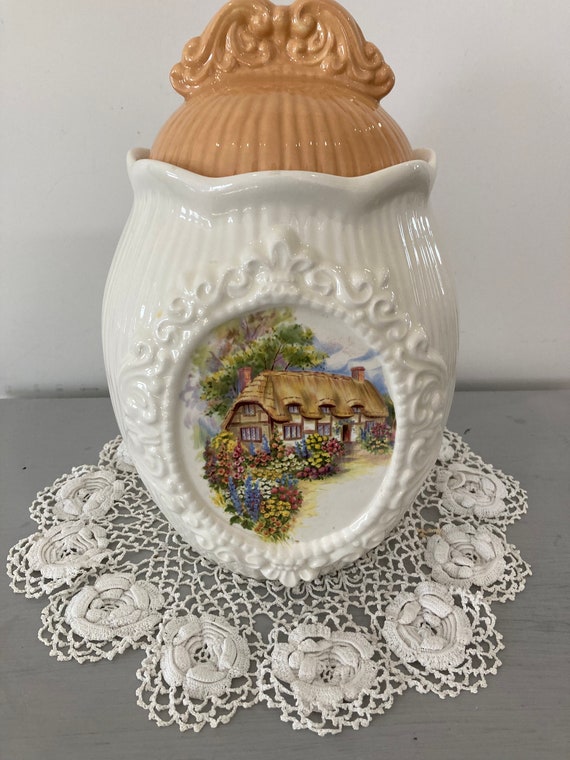This image presents an ornate, antique ceramic jar, reminiscent of an old-fashioned cookie jar, which is egg-shaped and rests atop a delicate, lace doily adorned with fabric roses in various colors arranged in a flower shape. The jar's base, predominantly white ceramic, features vertical ridges and intricate Celtic swirls. The front section boasts an ornate, fleur-de-lis-like garnish encircling a cut-out oval, showcasing a colorful and detailed painting of a quaint, Hansel and Gretel-style thatched house. This house has rose-colored shutters and an abundance of brightly colored flowers—roses, yellows, blues, and whites—at its front, complemented by a large tree in the background. About three-quarters up, the ceramic flares out and transitions into a peach, almost beige-ish, brown-ish orange ceramic lid with vertical ridges and an ornate crown-like decoration at the top, suggestive of a liftable lid. The entire ensemble sits on a grayish-painted wooden surface against a muted white background, imparting a nostalgic and timeless aesthetic to the scene.